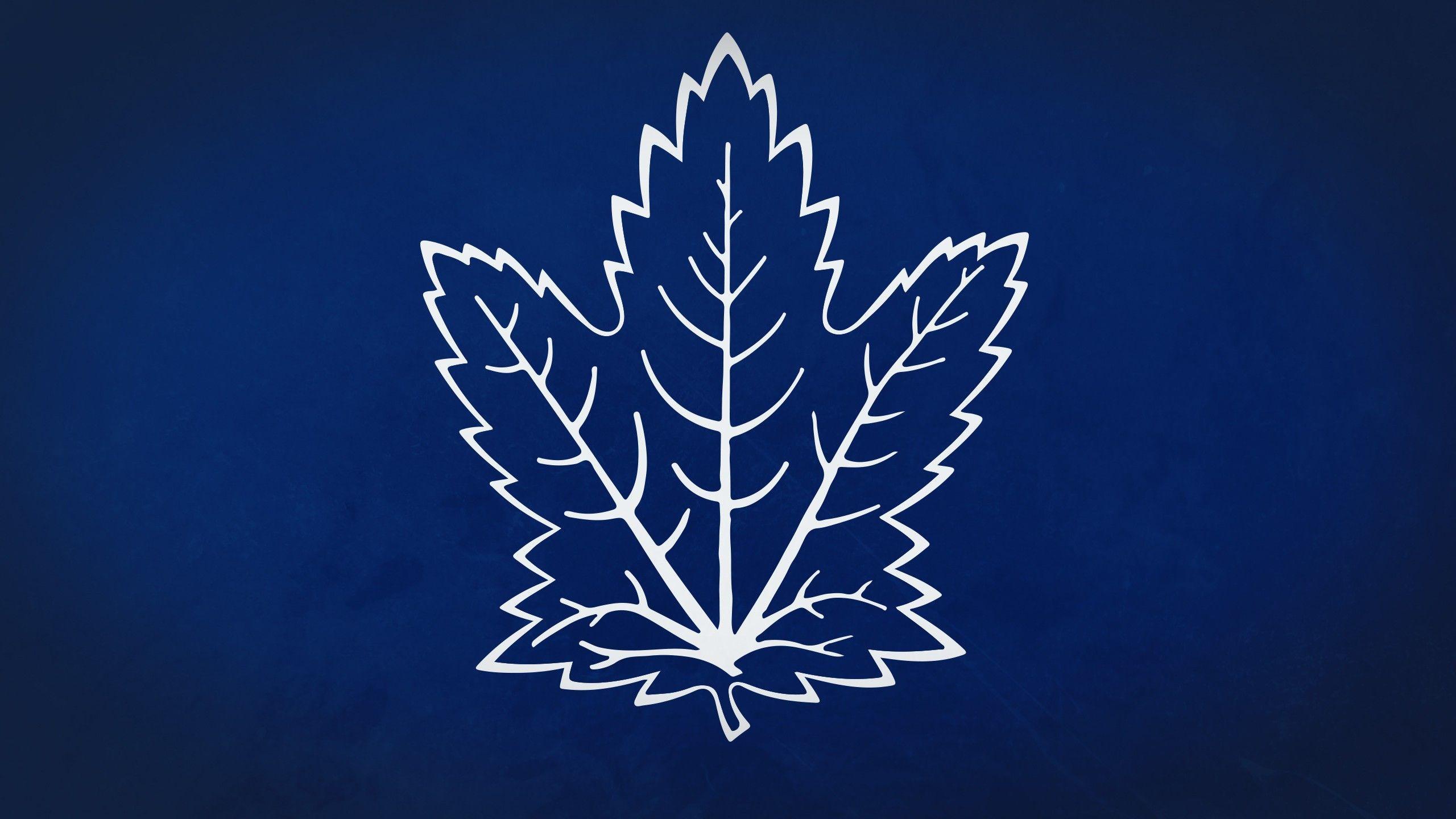The image features a detailed, artistic drawing of a leaf, prominently displayed in the center of a rectangular navy blue background that fades to a lighter blue in the middle. The leaf, outlined in white lines, is reminiscent of a maple leaf but with a unique structure that includes both three and five jagged points, resembling a star. Each section of the leaf and its edges are sharply defined with numerous spikes. The short stalk at the bottom of the leaf is also distinctly visible. Within the leaf, a pattern of vein-like lines creates a tree-like structure, adding to the artistic nature of the image. This design could remind viewers of the Toronto Maple Leafs logo or the leaf symbol on the Canadian flag.